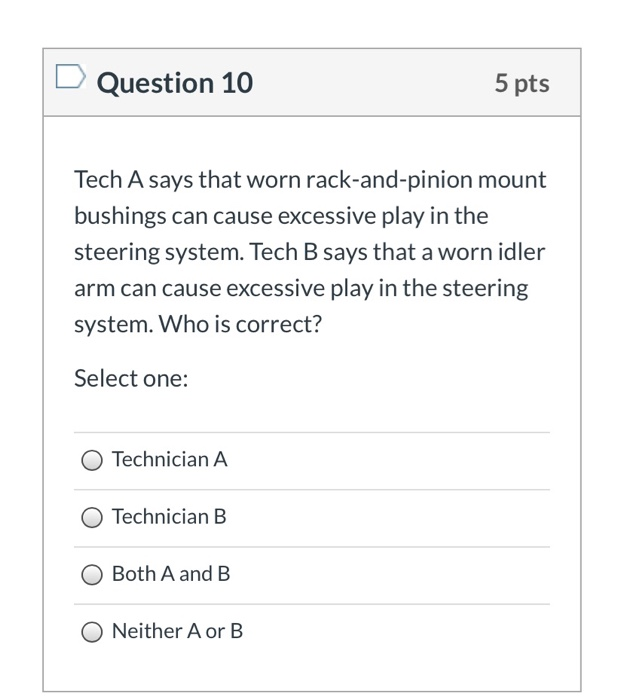The image showcases a test or survey question contained within a square box, featuring a detailed layout. The box itself is bordered and sits atop a light gray background. At the top of the box, there is a descriptive header with a price tag icon to its left, suggesting a formal or standardized format. This header states "Question 10" in bold letters, followed by "5 points" on the right in a similarly bold font.

Beneath this header, the actual question is displayed on a white background. The question reads: "Tech A says that worn rack and pinion mount bushings can cause excessive play in the steering system. Tech B says that a worn idler arm can cause excessive play in the steering system. Who is correct?" Below the question, the instruction "Select one:" is clearly written, followed by a colon.

The available answer choices are neatly listed with circular bullets for selection:
- Technician A
- Technician B
- Both A and B
- Neither A nor B

Each option is separated by a thin gray line for clarity, extending across the width of the selection area. The answer section concludes with a blank segment of the white background, providing a clean and organized presentation.